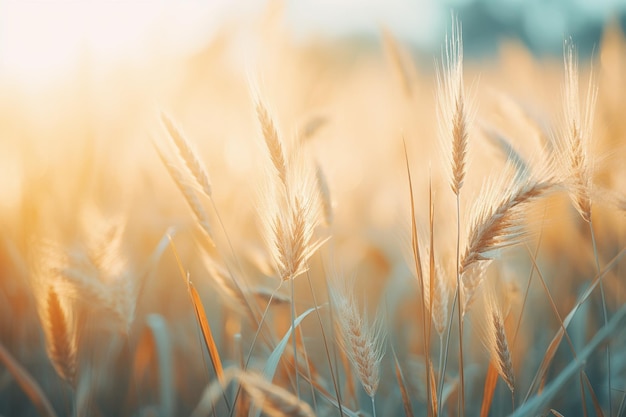A vast field stretches out, filled with what appears to be wheat, each stalk crowned with light brown tips that catch the sunlight. The wheat stands tall, reminiscent of grasses seen in arid regions. Despite the dry appearance, smaller green blades of grass peek through at the base, adding a touch of verdant life to the scene. The sun, positioned in the upper left of the image, bathes the field in a warm, golden light, highlighting the texture and color variations in the wheat stalks. This cultivated landscape captures the serene beauty of an agricultural expanse under the bright, inviting sun.